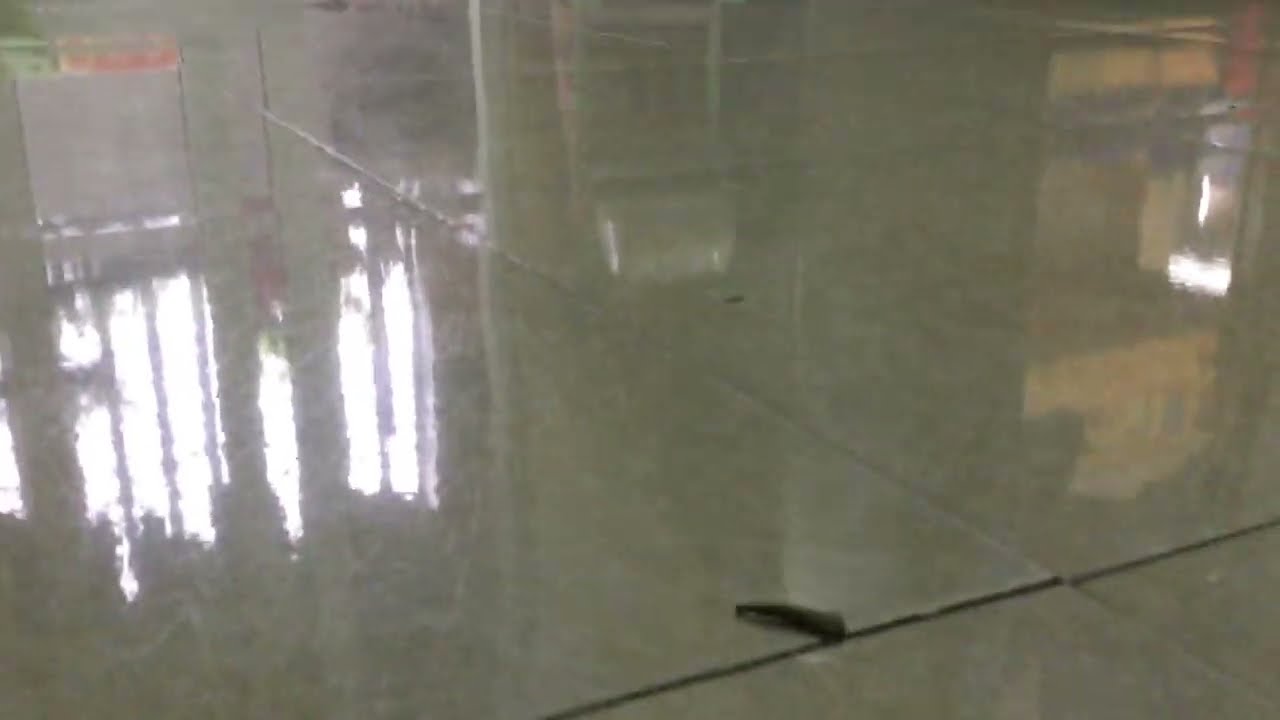This photograph captures a highly reflective, wet-looking floor, likely polished either from rain or water, creating vivid reflections. The pavement is tiled with large squares, incorporating both light and dark grout lines. Prominently in the lower center is an enigmatic small black or brown object, possibly a foot long, whose exact nature remains unclear—perhaps resembling a microphone or a remote. Reflective images play across the surface: on the left side, windows are reflected with sunlight streaming through, accompanied by what appears to be a fire extinguisher. The right side showcases a reflection of a possible yellow store. Dominating the center, white pillars and various lights are mirrored in the shine. Additionally, the top left corner introduces a splash of color with orange and green hues.